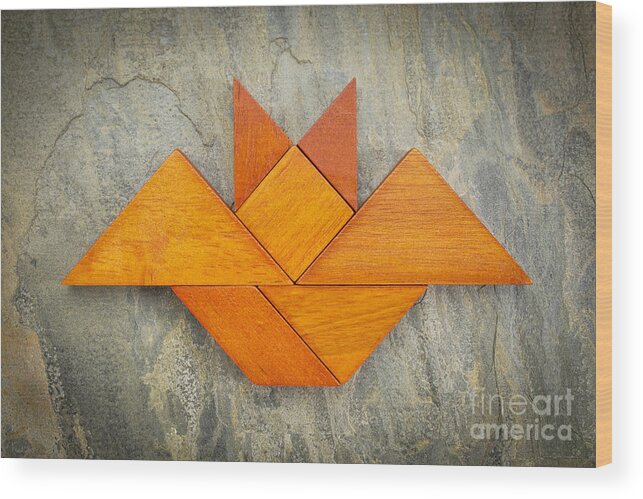The image depicts an abstract piece of art displayed on a textured, grayish-brown background that resembles concrete. The artwork is composed of various wooden shapes stained in shades of orange, yellow, and brown, arranged in an intricate, visually engaging pattern. The shapes include triangles, parallelograms, diamonds, and quadrilaterals, creating a complex geometric design. At the top, two triangles could be interpreted as ears or peaks, while additional triangles and diamonds below suggest lower facets or extensions of the form. This arrangement offers a dual interpretation, reminiscent of both a fox with pointy ears and wing-like extensions or an angelic figure. The dry brush blue effects on some of the wood pieces add a contrasting texture and color. In the bottom right corner, the phrase "fine art america" is superimposed in white lowercase font, subtly blending into the overall composition.